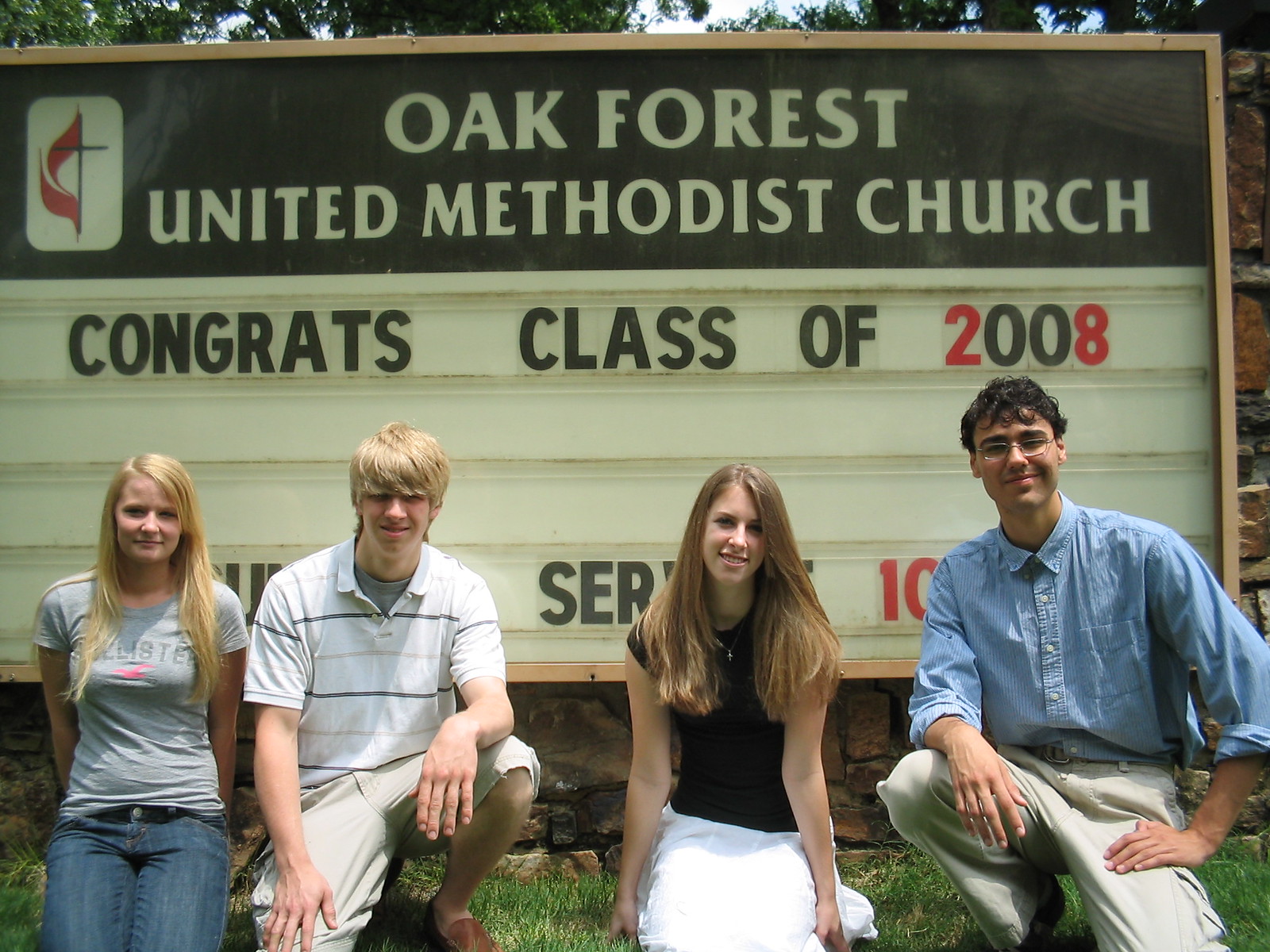This is a photograph taken on a sunny day, capturing four young people sitting on the grass in front of a church sign with green trees and patches of blue sky and clouds in the background. The sign reads "Oak Forest United Methodist Church" in white letters on a brown background, accompanied by a cross logo on the left. Below this, the sign has interchangeable letters spelling out "Congrats Class of 2008" in black and red. The group, likely high school graduates, consists of two young men and two young women. The woman on the far left has blonde hair, is wearing a gray t-shirt and jeans, and sits beside a man with blonde hair, dressed in a white shirt and beige shorts. Next to him is a woman with brown hair, dressed in a dark black top and a white skirt. The man on the far right wears a blue shirt, tan pants, and glasses. They are all staring directly at the camera, memorializing their graduation day.